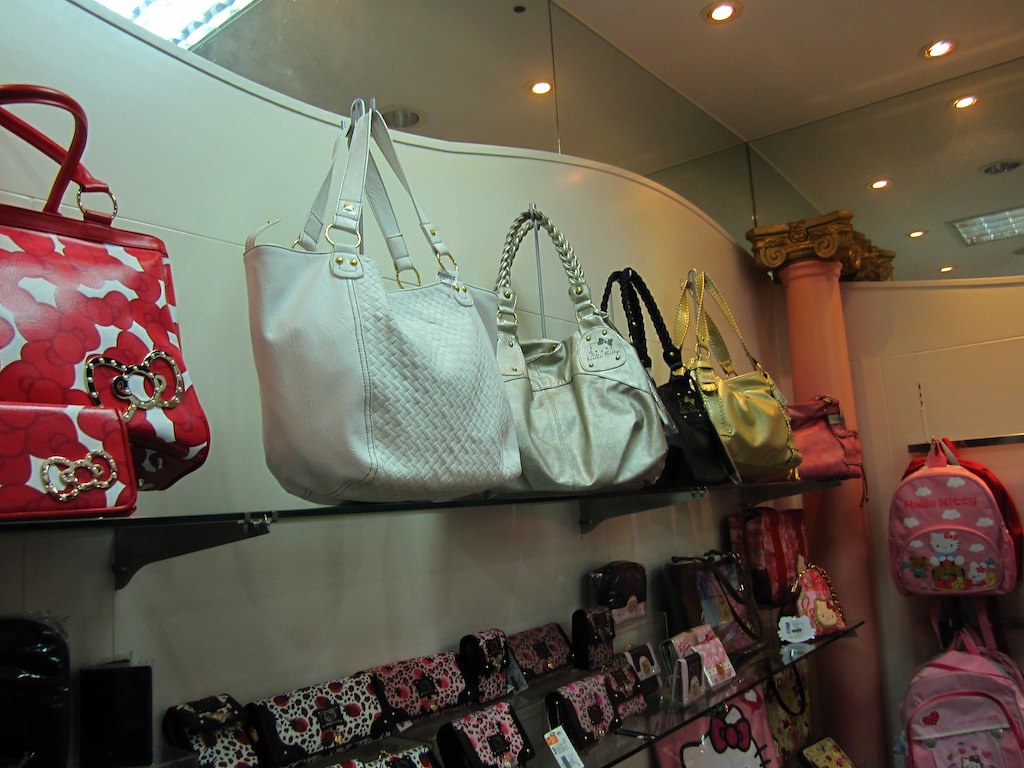The image is a color photograph of a store display within a shopping mall. The display consists of glass shelves arranged against a sleek, curvilinear white wall, adorned with a wooden Greek column featuring a curvy gold-carved Ionic or Doric capital. This backdrop highlights a collection of designer handbags. The top shelf prominently showcases fancy, large, and bulky handbags in various colored leathers, including a red and white patterned bag, two white purses, a black bag, a gold handbag, and a brown leather one. 

Beneath the handbags, the middle shelf is lined with smaller clutch purses that lack handles, available in various colors and prints. To the right of these shelves, in the far background, several children's backpacks are visible, including a notably recognizable Hello Kitty bag. The store features high ceilings with recessed lighting, and reflective surfaces, such as mirrored panels, that capture different angles of the space and enhance the store's modern, bright atmosphere.